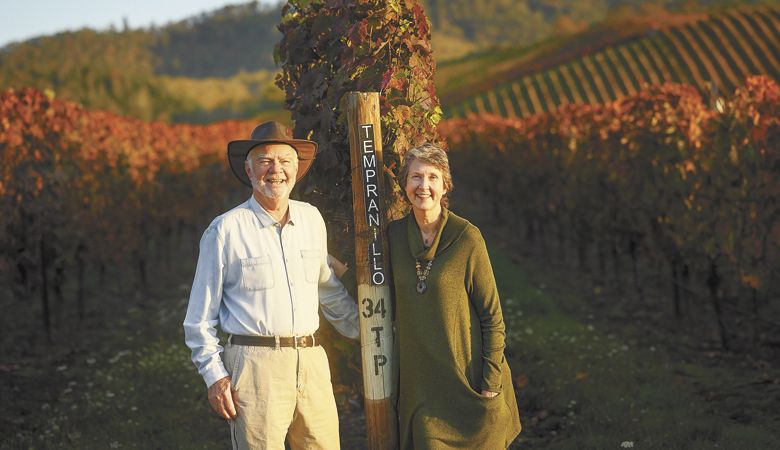The image depicts an older couple standing side by side, smiling at the camera amidst a vineyard. A wooden post between them prominently reads "TEMPRANILLO 34 TP" in black lettering, with some parts painted white. The man on the left sports a brown cowboy hat, a light blue button-down shirt, khaki pants with a black belt, and has a thin gray beard. The woman on the right, with short, wavy gray hair, is dressed in a long green sweater or dress, a necklace, and has her hand in her pocket. Behind them stretches a picturesque vineyard with rows of grapevines bearing orange-red leaves, set against a backdrop of a distant mountain range under a light blue sky. The colors of the vineyard, however, appear slightly off, giving the image an almost inverted hue effect.